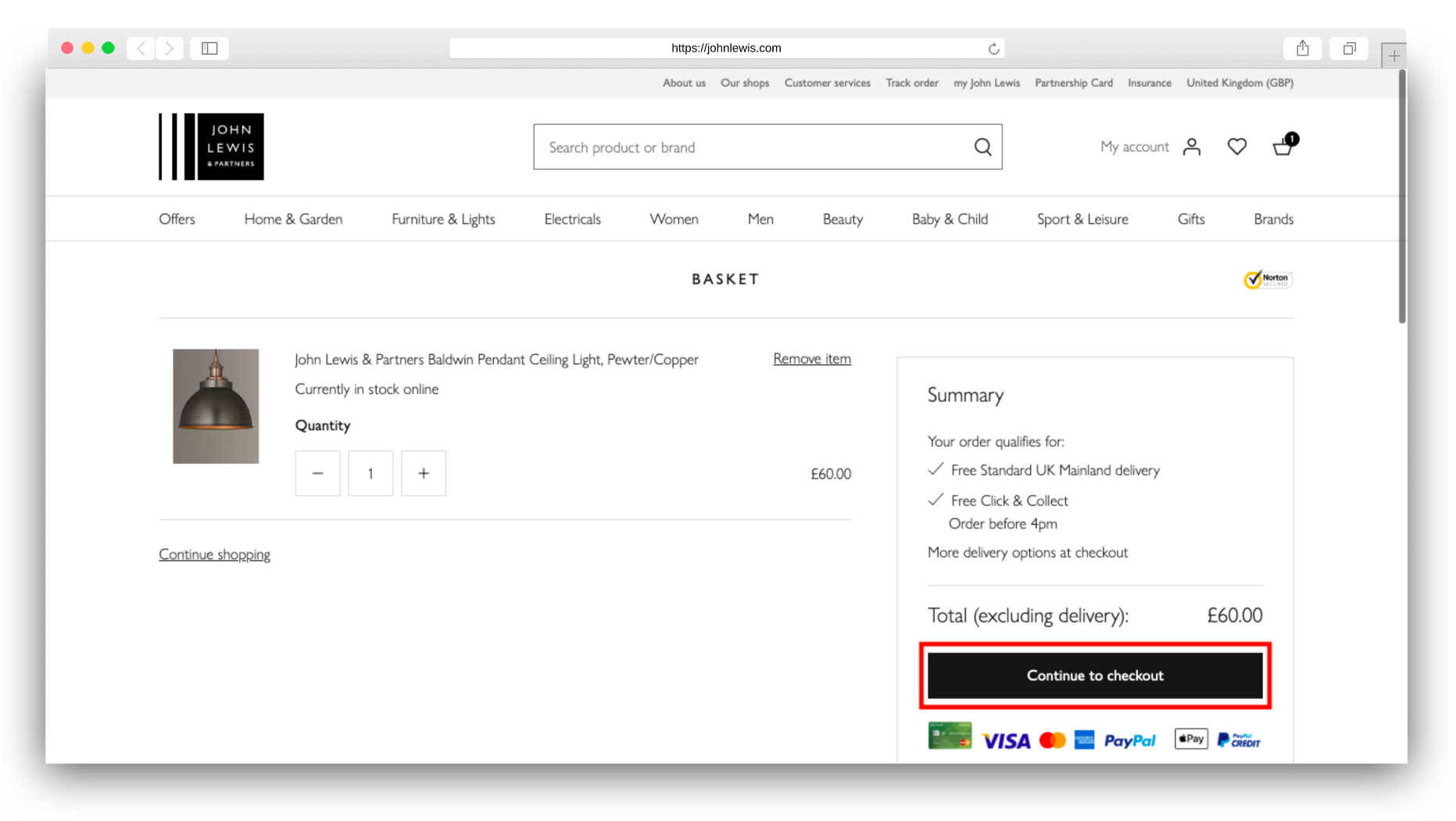A shopper at John Lewis has placed a striking copper overhead lamp in their basket, priced at $60. The elegant design suggests it is more suitable for a commercial setting, such as a trendy wine bar, rather than a home environment. The choice might reflect the shopper's ambition to start a new business, perhaps a wine bar, as a significant personal venture. They seem ready to make this investment to bring their entrepreneurial vision to life.